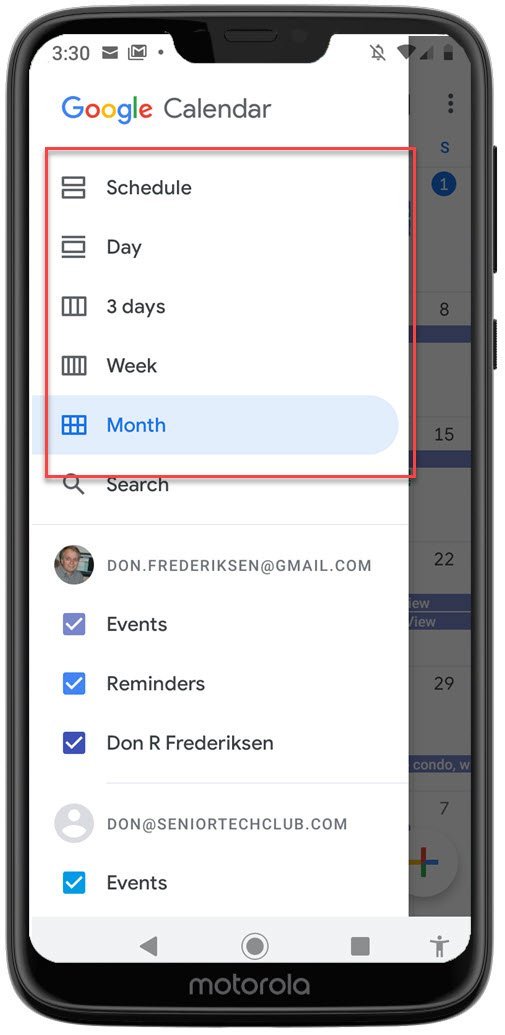The image depicts an iPhone with a black exterior frame, displayed in portrait orientation, showing the home screen. The time reads 3:30. The status bar at the top includes several icons: an envelope symbol, a square with the letter "M" inside, a bell with a line through it indicating silent mode, a Wi-Fi signal, a cellular signal indicator, and a battery icon.

Prominently displayed is the Google Calendar interface. The right side of the screen shows a dark gray overlay that vertically runs from the top to a portion of the display. Within the Google Calendar app, various navigation tabs are visible: "Schedule," "Day," "3 Days," "Week," and "Month." The "Month" tab is currently selected, highlighted in a blue banner with blue text.

Below this, there is a search bar with "Don.Fredrickson@gmail.com" typed into it. Below the search bar, the interface lists "Events" and "Reminders," followed by the account name "Don R. Fredrickson." Additionally, it mentions another account, "Don at SeniorTechClub.com", along with its associated events.